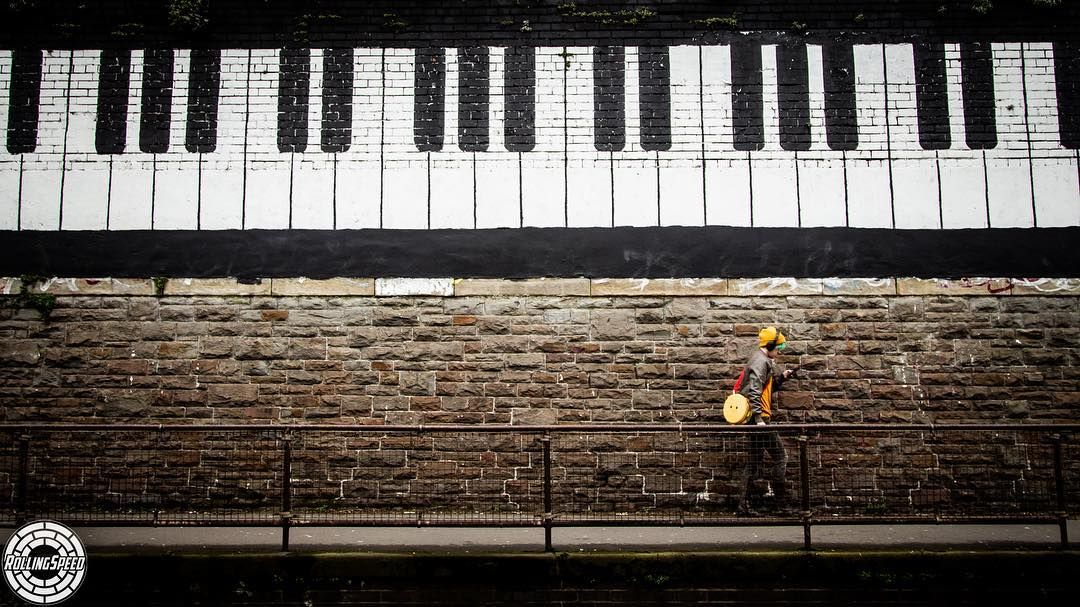A pedestrian strolls along a red and brown brick sidewalk adjacent to a building adorned with a massive mural. The mural, occupying the upper half of the structure, depicts a piano keyboard complete with prominent black and white keys framed by thick, black lines. In the bottom left corner of the image, a white, circular sewage cap branded with the "Rolling Speed" logo is visible, adding an unexpected element to the urban landscape. The individual in focus sports a vivid yellow winter cap and carries a matching yellow circular purse. They are clad in a brown leather jacket, complemented by gray jeans and sturdy, gray boots, exuding a chic, yet practical winter style.